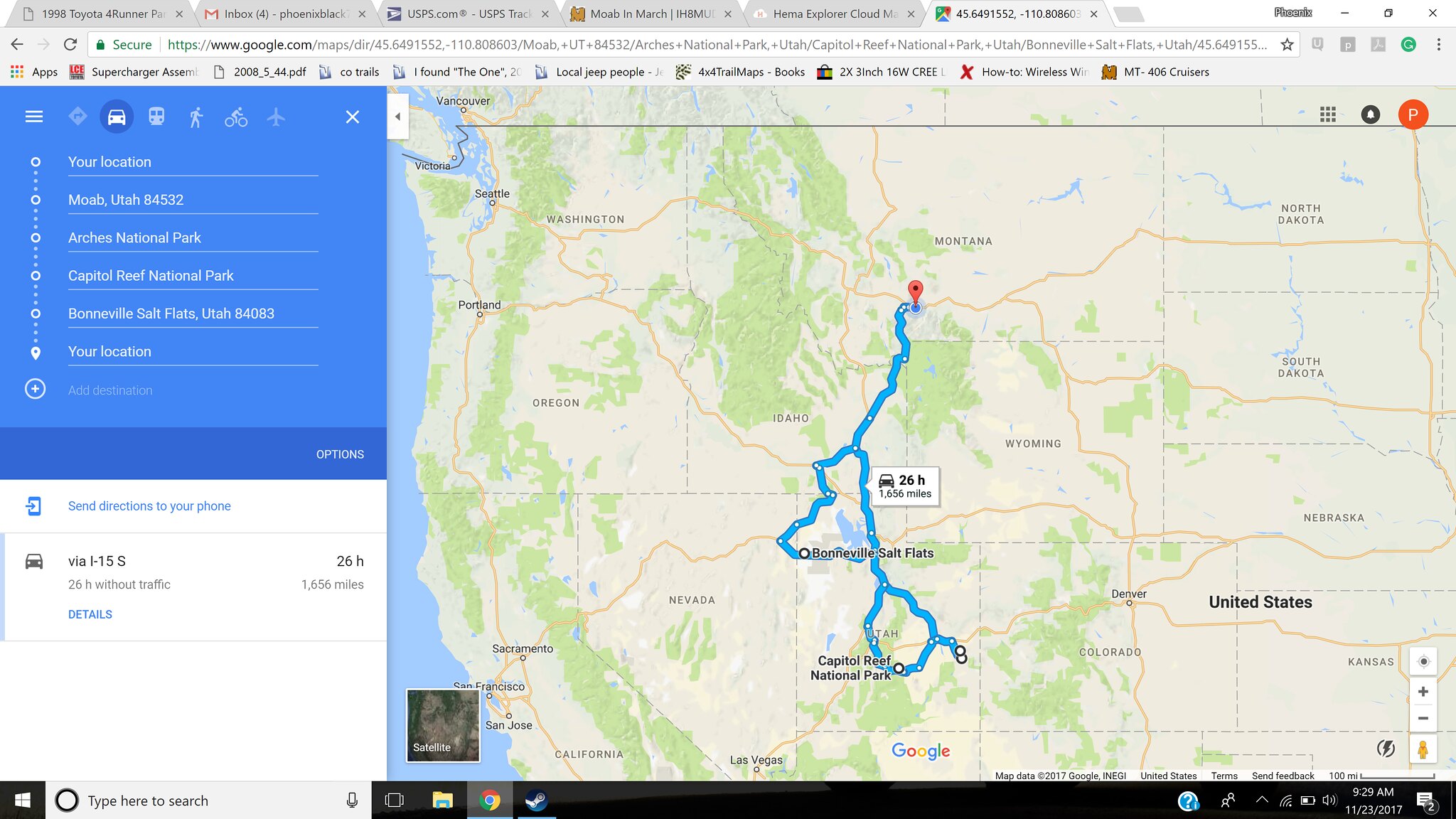This image captures a screenshot from a computer browser, likely Microsoft Edge, displaying Google Maps. The central focus is a detailed map of the Western United States, prominently showcasing a driving route highlighted in blue. The journey, extending 1,656 miles, is estimated to take 26 hours via I-15 South. The route begins at the border of Montana and stretches down to Capitol Reef National Park in Utah, passing landmarks such as Moab, Utah, Arches National Park, Bonneville Salt Flats, and Capitol Reef National Park. The map occupies approximately 80% of the screen, with the remaining space displaying standard browser elements, such as six tabs at the top and the web address. The top left features a blue box with driving instructions and key details about the route.